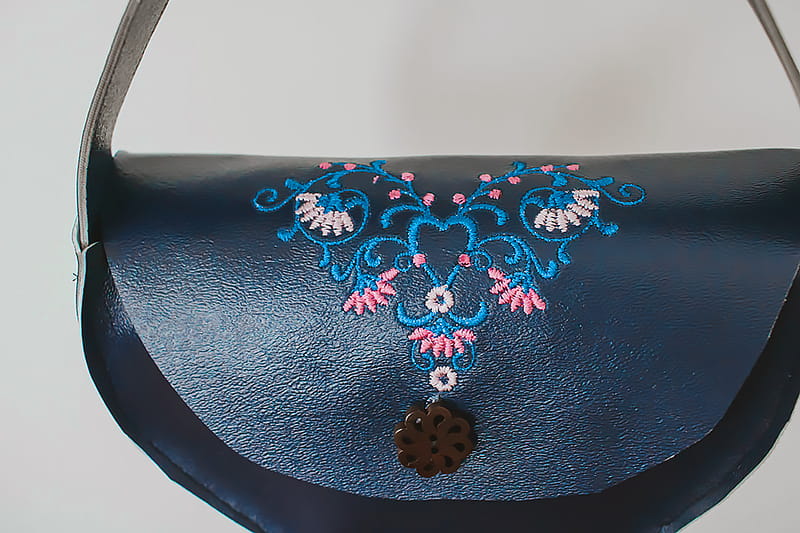This image features a handcrafted dark blue purse made from a shiny pleather material reminiscent of car upholstery. The purse has a thick strap, making it suitable as a shoulder bag, and it possesses a unique crescent-shaped body. The flap of the purse, though slightly misshapen on one side due to uneven cutting, adds to its handmade charm. The most striking element of the purse is its detailed embroidery located above the button closure. The button is brown, circular, and has a swirled texture. The embroidery above it features an intricate design: a blue heart from which a blue vine with little pink and white flowers emerges. This vine mirrors on both sides of the heart, ending with alternating larger pink and white flowers. The bag is photographed on a white surface, though the bottom and the right side of the purse are slightly cut out of the image frame. The overall aesthetic, with its vivid blue, pink, and white floral pattern, gives the purse an appealing, high-end boutique feel.